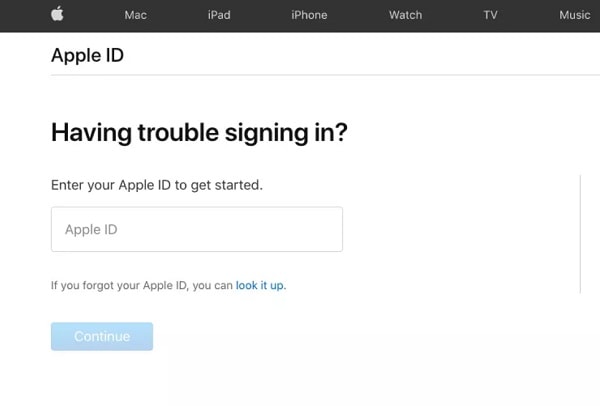The image depicts the Apple website, focusing primarily on the Apple ID sign-in page. At the top of the image, there is a black navigation bar featuring several icons and tabs. On the left side of the bar, the silver Apple logo is prominently displayed. Moving right, there are tabs labeled "Mac," "iPad," "iPhone," "Watch," "TV," and "Music."

Below the black navigation bar, the background transitions to white. In the upper left corner, "Apple ID" is displayed in bold black letters. Underneath "Apple ID," a thin light gray line separates it from the rest of the content.

Further down, bold black text poses the question, "Having trouble signing in?" Directly below this question, instructions read: "Enter your Apple ID to get started," accompanied by an empty input box where users can type their Apple ID. Below this box, guidance text states, "If you forgot your Apple ID, you can look it up," with "look it up" being a clickable hyperlink. At the bottom of this section, there is a blue "Continue" button.